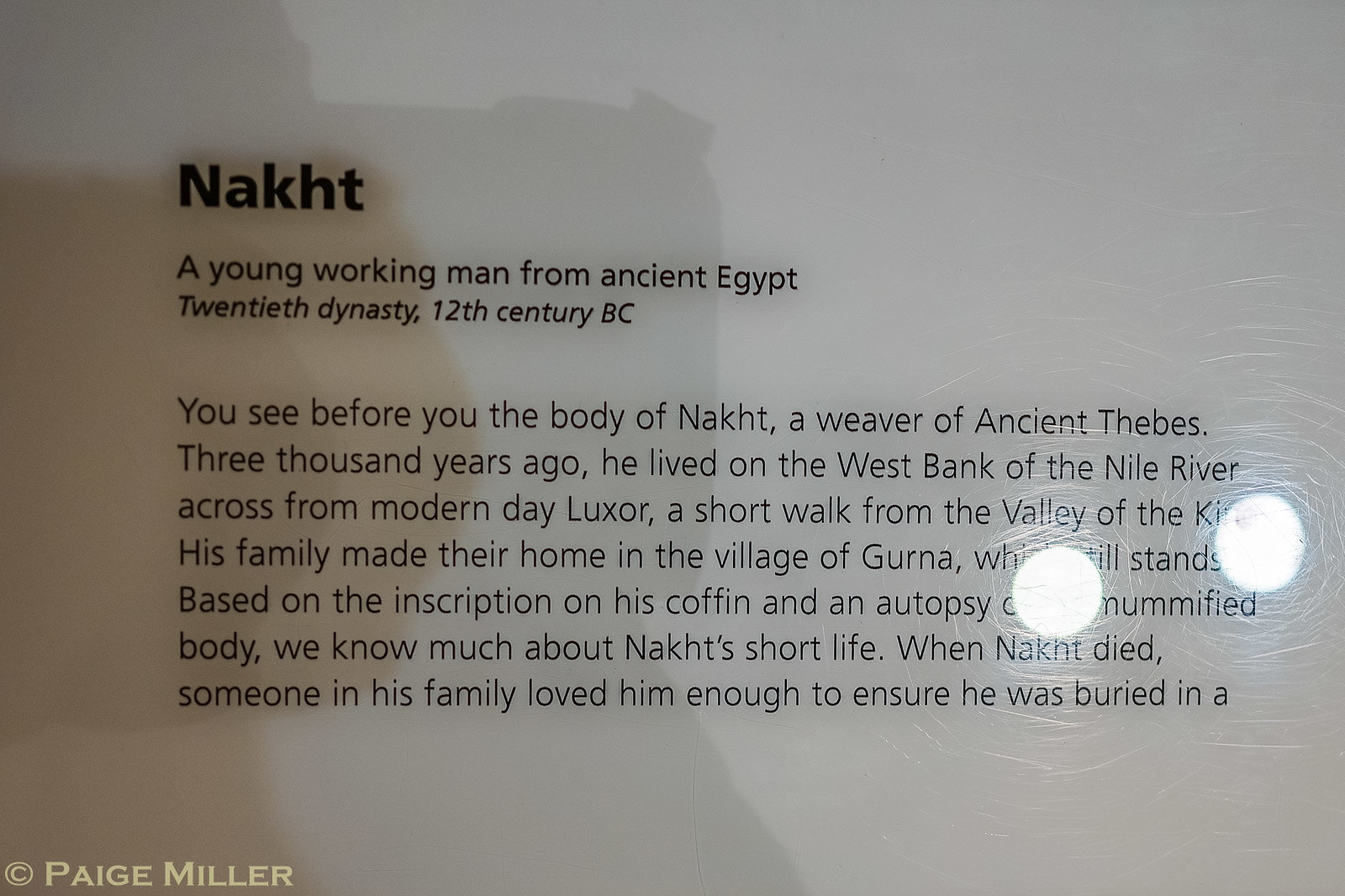The image captures a highly reflective informational plaque, possibly made of plastic or acrylic, displaying detailed historical information. The plaque prominently features the name "NAKHT," spelled out in large, bold black letters at the top. Below, it introduces Nakht as "a young working man from ancient Egypt, 20th dynasty, 12th century BC." Further down, you learn more about his life: "You see before you the body of Nakht, a weaver of ancient Thebes." Additional text elaborates that Nakht lived on the west bank of the Nile River, near what we now call Luxor, and his family resided in the village of Gurna, which still exists today. The plaque's background is white with multiple lines of black text, and two lights are reflected on the right side of the image. The shadow of the photographer is visible on the left, and a yellow font inscription on the bottom left reads "© Paige Miller."